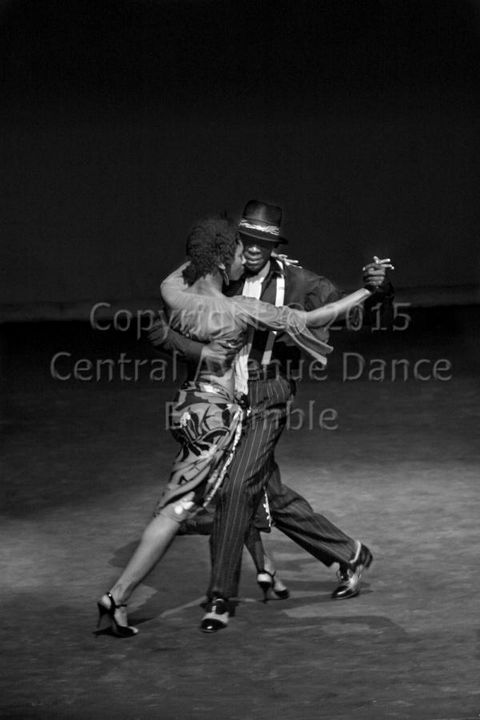This is a black and white photograph featuring an African-American man and woman dancing together on a dimly lit stage, likely as part of a performance by the Central Avenue Dance Ensemble, as indicated by the "Copyright 2015, Central Avenue Dance Ensemble" watermark overlaying the image. The couple, illuminated by a spotlight that forms an oval shape on the floor around them, appears to be performing an Argentine tango. The man, positioned to the right in the frame, wears a black bowler-style hat, a black suit with a white undershirt, black pinstripe pants, white suspenders, and polished dance shoes. The woman, who is closer to the camera and slightly turned away, is dressed in a dark, floral-patterned skirt and black high heels. She has short-styled hair and wears an earring. The pair is intimately embraced with the man's right arm around the woman's back, while their left hands are clasped together, indicating a tight, cohesive dance posture. The stage, otherwise shrouded in darkness, focuses all attention on the dancers and their period-evocative attire, lending a timeless, classic atmosphere to the scene.